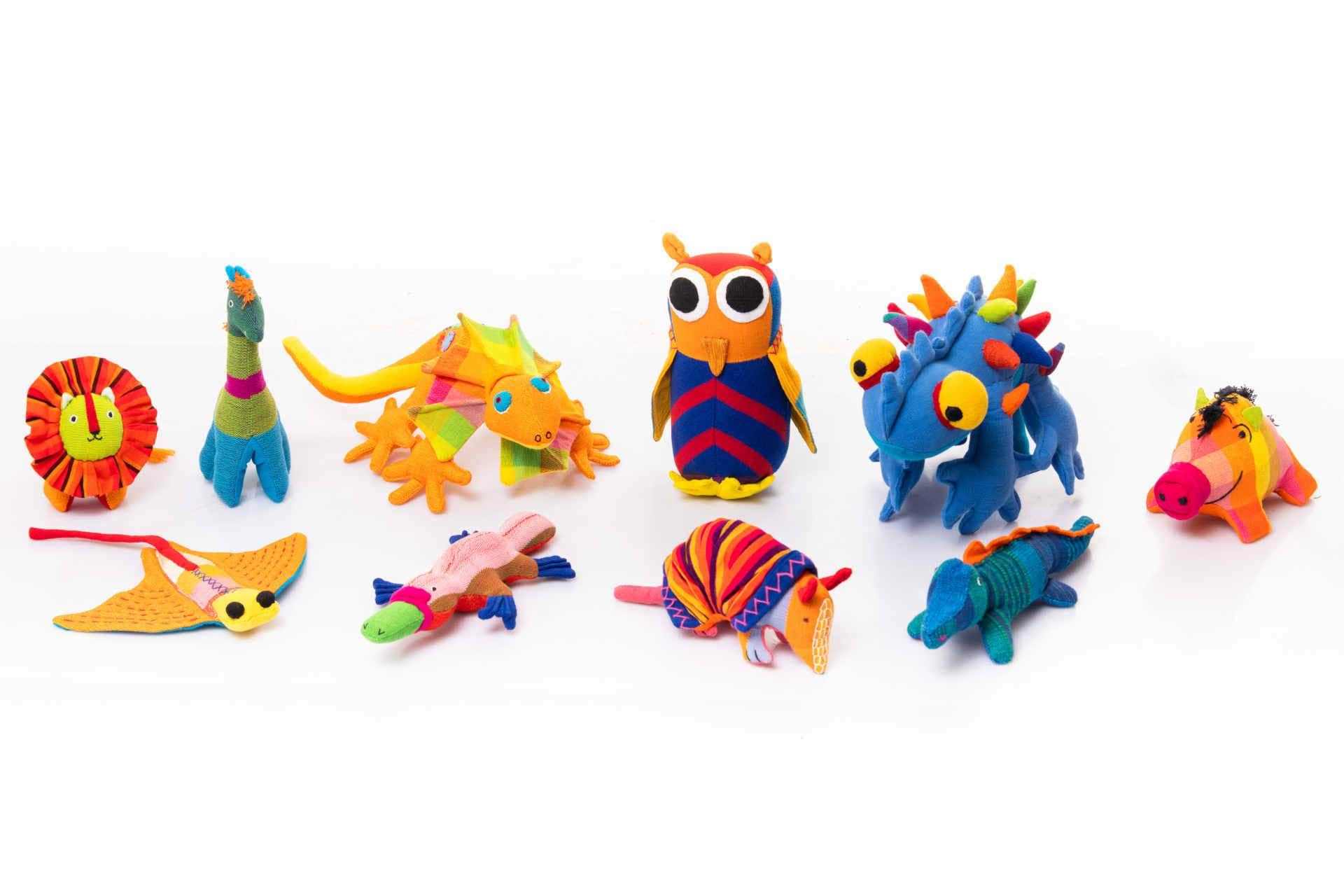In this vibrant and whimsical scene, ten plush toys are arranged against a stark white backdrop, drawing attention to their colorful designs. The toys, made from a soft, felt-like material and stuffed for a plush feel, are arranged in two rows with smaller animals in the front and larger ones in the back. In the back row, starting from the left, there's an orange lion, followed by a blue giraffe. Next is a yellow dinosaur-like creature, a blue and orange owl, an indeterminately shaped blue creature with colorful spikes, and a pig-like figure on the far right. In the front row, beginning from the left, we see a yellow stingray, a brown and pink platypus, a red, blue, and dark brown armadillo, and finally, a small blue dinosaur. Each toy showcases a combination of bright hues, predominantly orange, yellow, and blue, making them visually appealing to young children, likely targeting an age range of two to four. Their whimsical and imaginative designs give a playful twist to familiar animal forms.